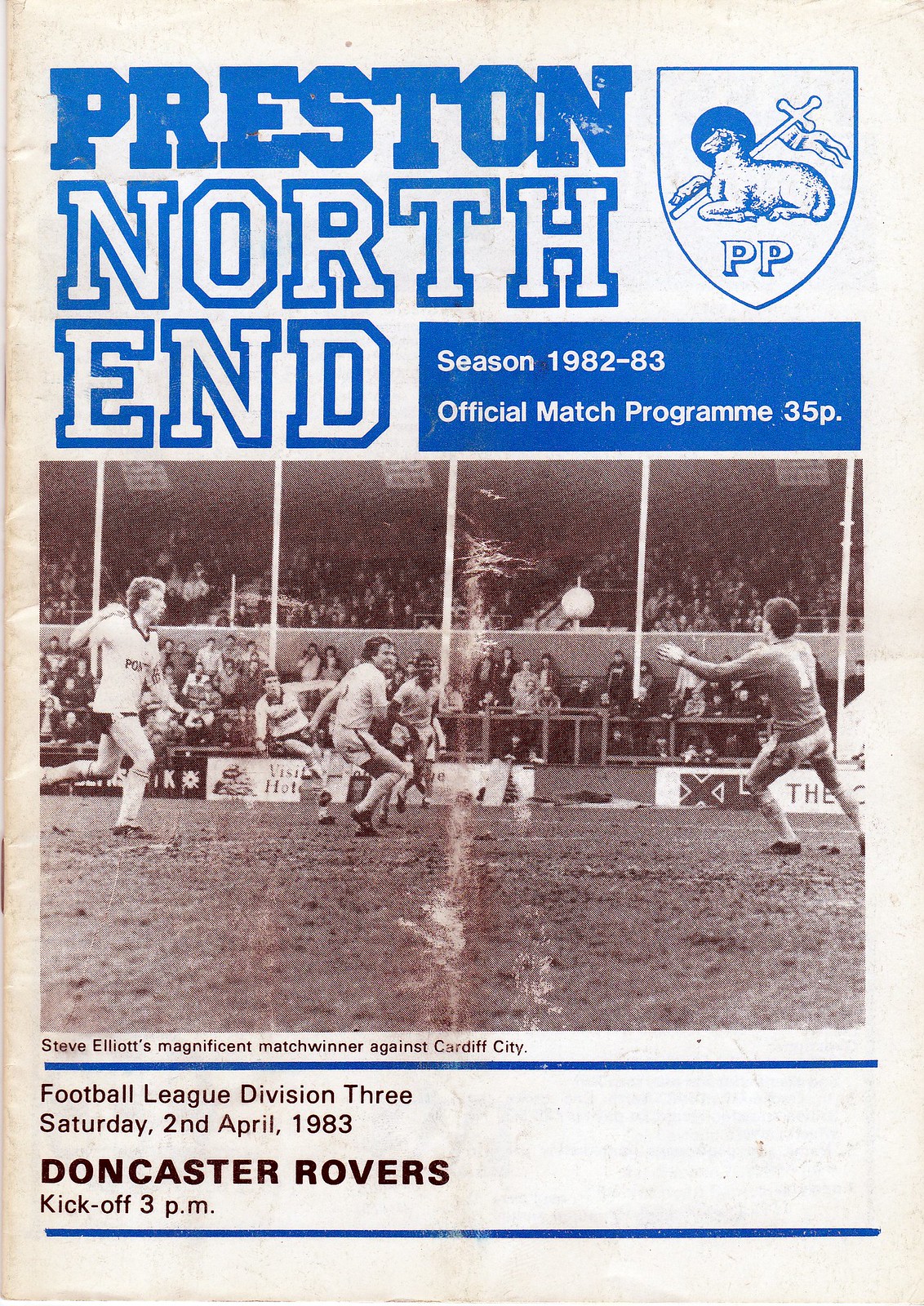The cover of the sports team's program is on white paper. At the very top, in blue text, it reads "Preston," followed by "North End" in white text with blue borders directly underneath. To the right of these titles, a blue rectangle contains the white text: "Season 1982-83 Official Match Program 35P." In the top right corner, above this rectangle, there is a white shield shape with a blue border displaying a lamb laying down and holding a flag, with the letters "PP" in white and blue borders inside the shield. Dominating the center of the cover is a black-and-white photograph of a soccer game in progress, featuring several players on the field with the ball in midair. Below the photograph, there is black text detailing Steve Elliott's Magnificent Match Winner Against Cardiff City, Football League Division III, and the match information: Doncaster Rovers, Saturday 2nd April 1983, kickoff at 3 PM.